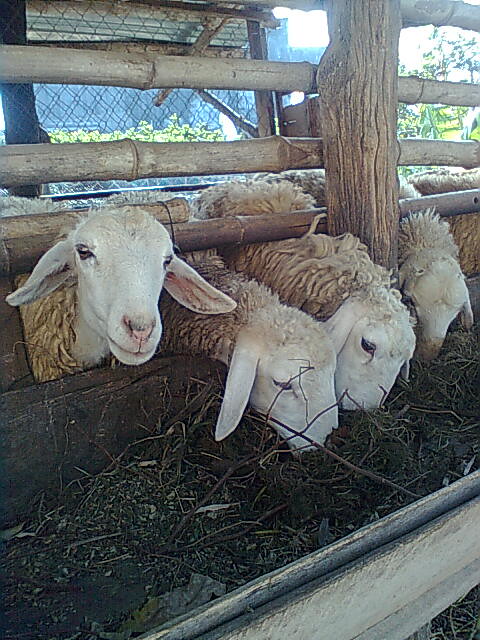The image captures four sheep in a pen, set against a bright daytime sky with some visible greenery in the background. At the top of the image, a wooden fence with long pillars and horizontal slats forms the primary barrier, while a secondary blackish metal fence with vertical diamond shapes is visible behind it on the left. The pen structure allows the sheep to poke their heads through the wooden slats to reach a trough filled with black, twiggy-like food outside the pen. Three sheep, located in the right middle section of the image, have their faces immersed in the trough, busily eating. One sheep, positioned towards the left middle, stands out by looking directly at the camera with a white face, a pink nose, black eyes, and floppy ears. This detailed scene highlights a typical, serene rural setting with the sheep seemingly enjoying their meal amidst their pen.